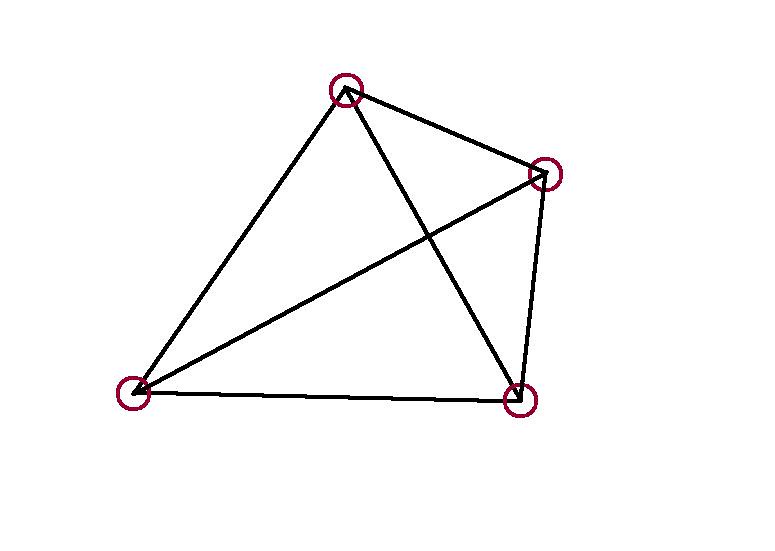The image features a kite against a white background. The kite, appearing to be digitally drawn, is oriented approximately 90 degrees to the right, giving it the appearance of lying down rather than standing upright. The kite's structure is defined by black, medium-thin lines forming a shape typical of kites: a larger triangle at the bottom connected to a smaller triangle at the top. A single line runs from the top left to the bottom right, accentuating its angled position.

At each of the four corners of the kite, there are outlined red circles. While most of the black lines are straight, the lines near the bottom right and very bottom corners exhibit slight crookedness, adding a subtle zigzag quality to the otherwise straight edges. The overall composition suggests precise, computer-generated lines except for the minor imperfections mentioned.